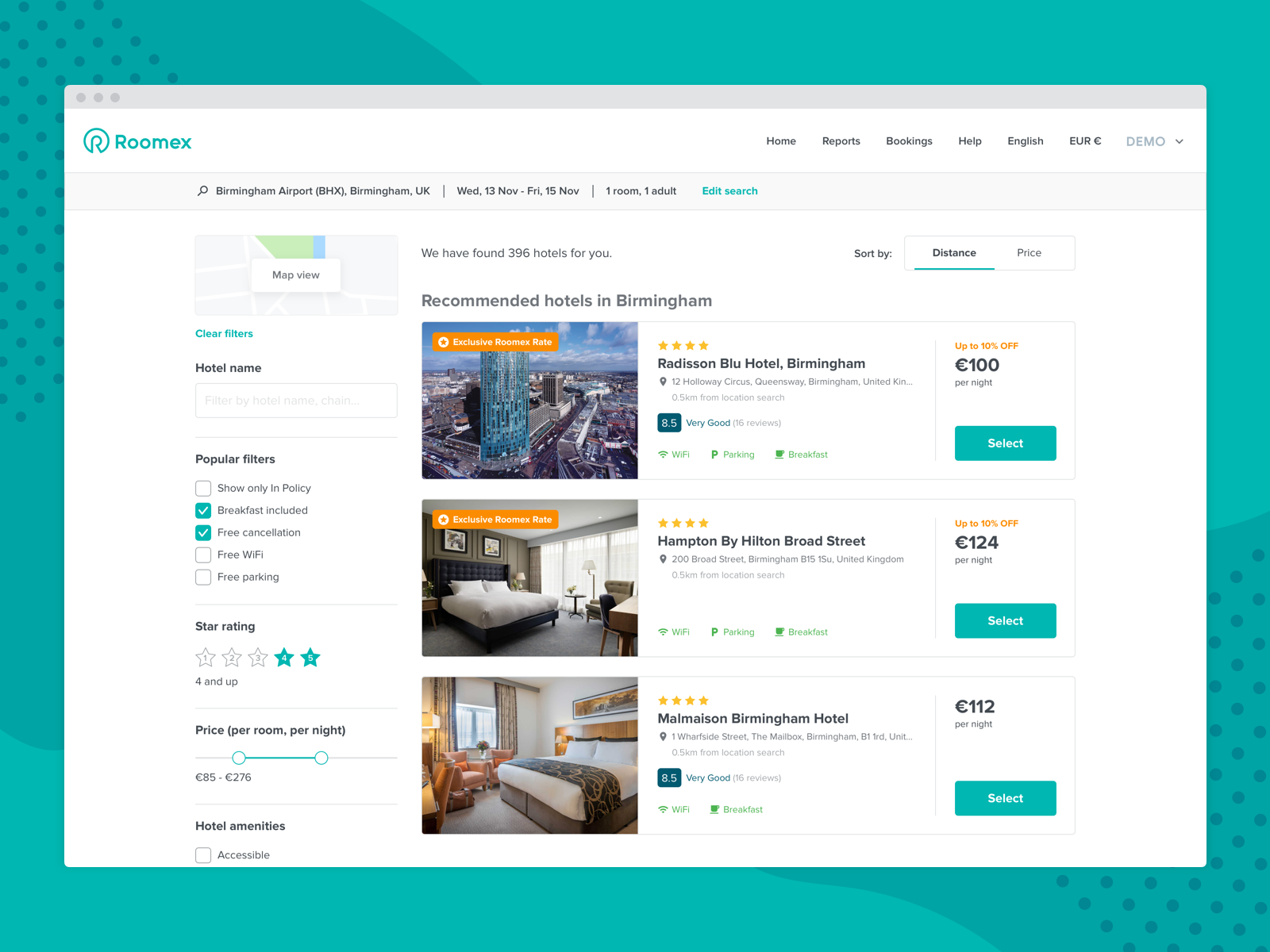The web page for RoomEx (R-O-O-M-E-X) features a teal blue background adorned with a polka dot pattern. Overlaying this background is a primary white content area that contains the main elements of the page. At the top of this white content area, a thin gray ribbon is followed by a wider white ribbon. On the left side of this ribbon, the word "RoomEx" is displayed in bright blue alongside its logo, an open circle. On the right side of the ribbon, several navigation options are listed in small gray text: "Home," "Reports," "Bookings," "Help," "English," "Euro," and "Demo" with a drop-down arrow.

Beneath this white ribbon, another thin gray ribbon appears, featuring a magnifying glass icon on the left for search functionality. To the right, the text reads: "Birmingham Airport, Birmingham, UK, Wednesday, 13 November to Friday, 15 November, one room, one adult," followed by a bright blue "Edit Search" option.

On the left side of the page, a vertical column provides filters for refining search results. At the top of this column, a small rectangular box displays a map with a "Map View" button. Below, a bright blue "Clear Filters" option stands out. Under this, the filter options include:

- "Hotel Name" with a box for entering the name
- Various filter criteria, including "Show Only in Policy," "Breakfast Included," "Free Cancellation," "Free Wi-Fi," and "Free Parking," with "Breakfast Included" and "Free Cancellation" being selected (indicated by bright blue checkboxes with white checkmarks)
- A star rating filter set to four stars and above
- A price range filter showing 85 to 276 pounds per room per night

The main content area highlights a section titled "Recommended Hotels in Birmingham" in bold gray text. Below this header, three hotel options are displayed vertically, each featuring an image, price, and star rating.